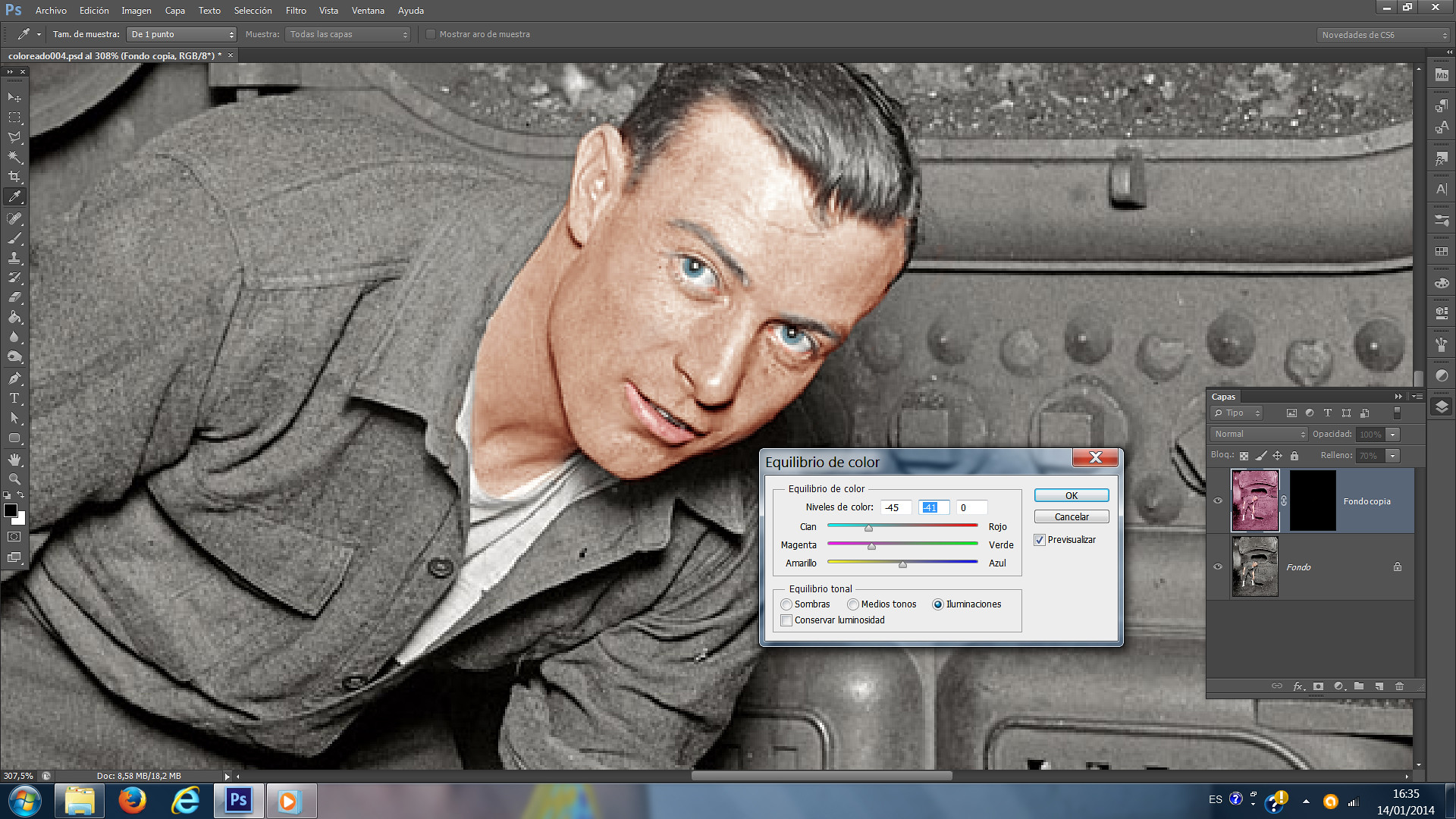This detailed caption synthesizes the shared and emphasized aspects from each contribution:

The image is a screenshot from a Windows computer, displaying a drawn depiction of a man. The computer screen's background is gray with a blue border at the top, and several icons are visible at the bottom, indicating possible use of an editing program like Photoshop or Paint. The man in the image is a white male with gray hair combed back, light blue eyes, and a half-smile showing his upper teeth. He appears to be bent over, wearing a gray collared shirt with buttons and a pocket on the left side, gray pants, and a white t-shirt underneath. His attire and overall appearance suggest he might be from the WWII era, perhaps in his 20s or 30s. The background includes a sign with illegible gray print on a white background, written in a different language. The overall effect of the colors might be influenced by the use of the color panel in the editing software.